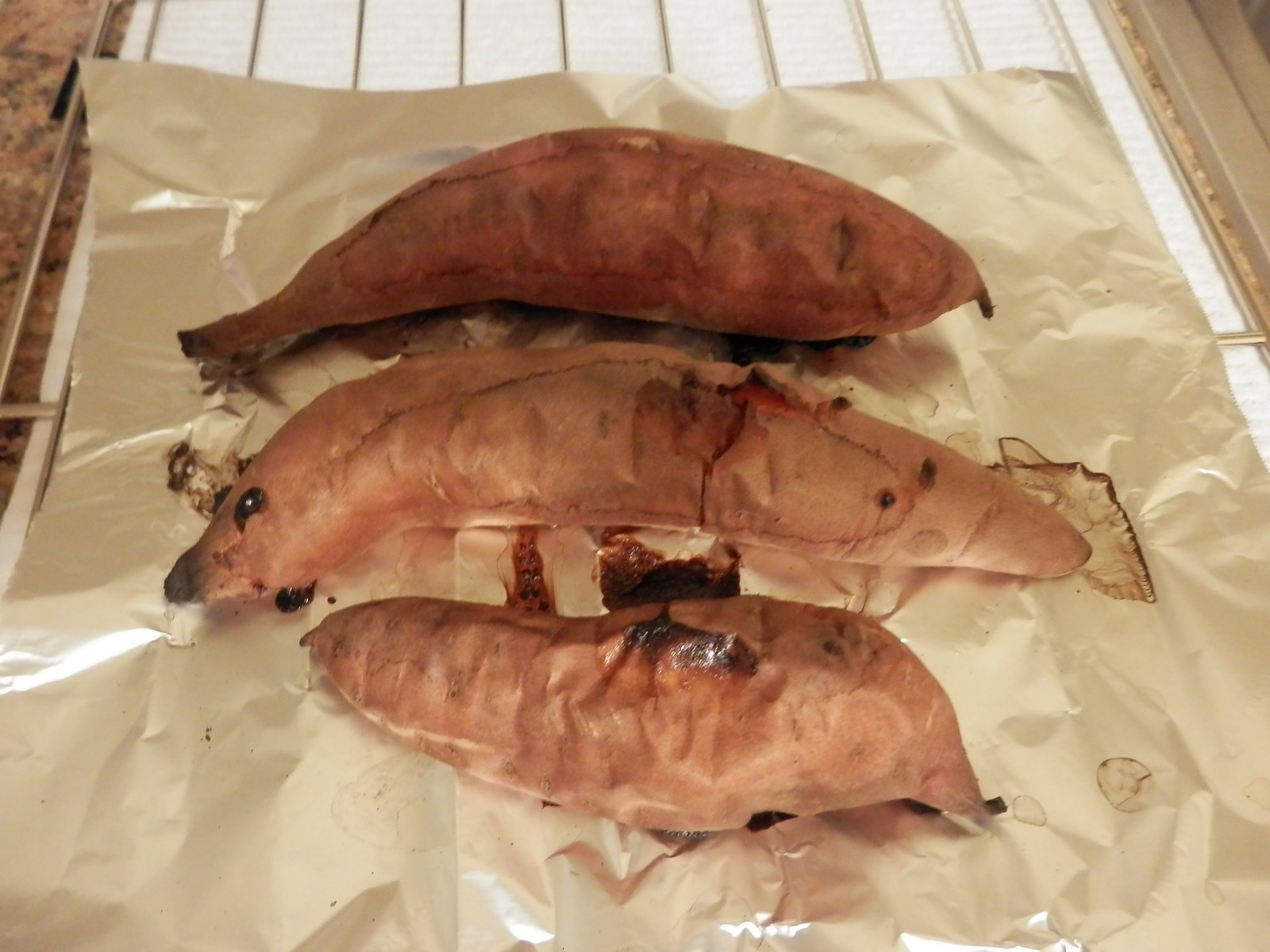The image showcases three freshly baked sweet potatoes resting on a large sheet of aluminum foil, which has a matte, yet reflective, silver metallic finish. The foil sits atop a metallic oven rack, characterized by several prongs that create a vented surface. The sweet potatoes are oblong and irregularly shaped, with pinkish-brown skins that exhibit a wrinkled texture and dark brown caramelization spots from the cooking process. One can also see a dark brown splatter of burnt sweet potato juice on the foil. The foil and rack are placed on a granite kitchen counter, which is primarily dark brown with lighter brown and beige tones. The scene indicates that the sweet potatoes have just been taken out of the oven and are ready for further preparation.